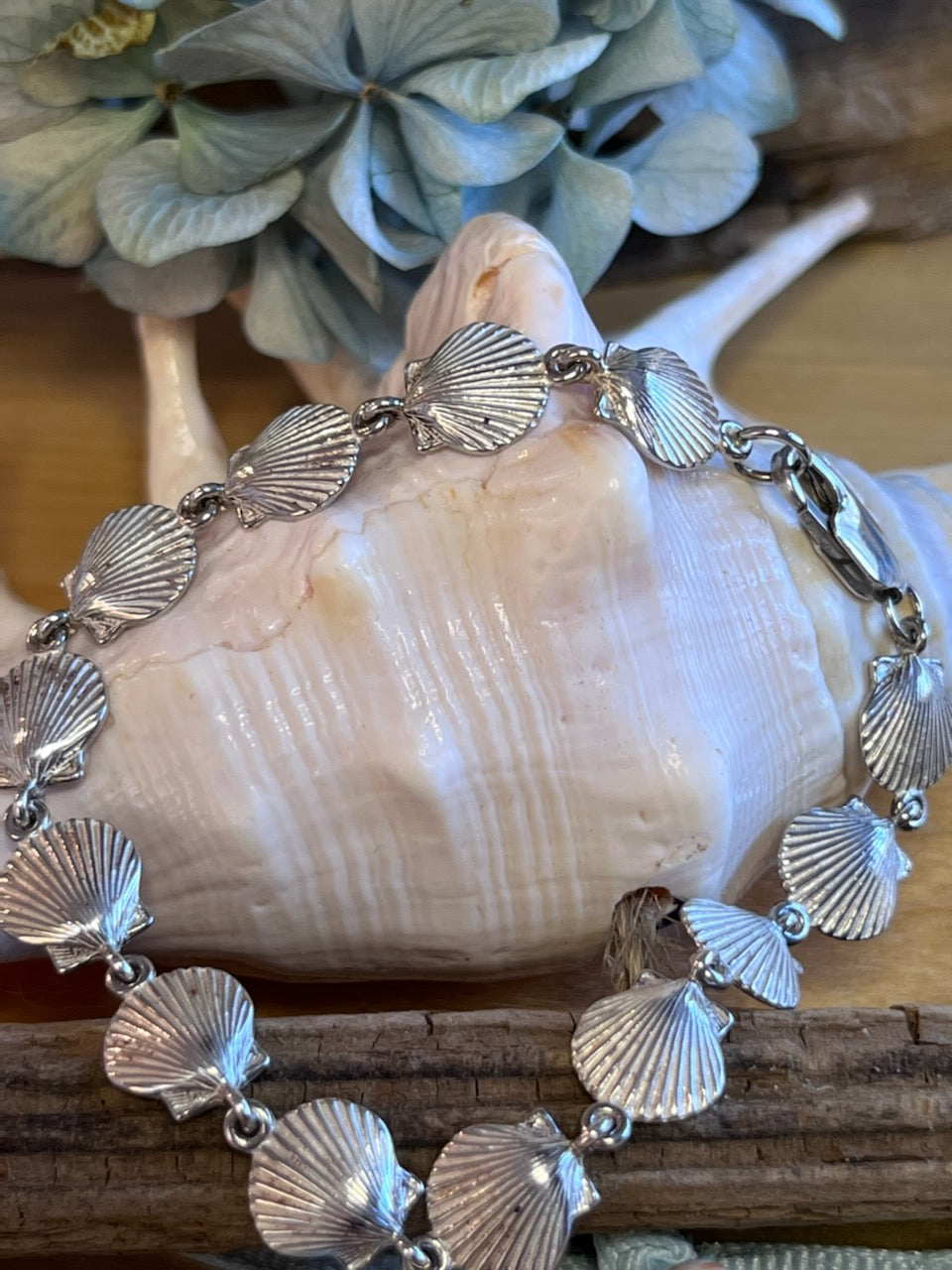This photograph, captured indoors, features a detailed composition centered around a large, shiny, oval seashell that ranges in color from pink to tan with delicate vertical stripes. The seashell dominates the center of the image, extending from the left across to the upper right-hand section, and is set on a worn brown wooden table. Draped over the seashell is a bracelet fashioned from approximately 14 to 20 small, pewter or silver shells, distinguished by a circular hook and a visible clasp on the right. Above the seashell, light green leaves and an assortment of bluish-gray flower petals cascade, adding a natural touch to the scene. In the foreground, the edge of the wooden table, possibly reminiscent of tree bark, underscores the rustic ambiance of the photograph.